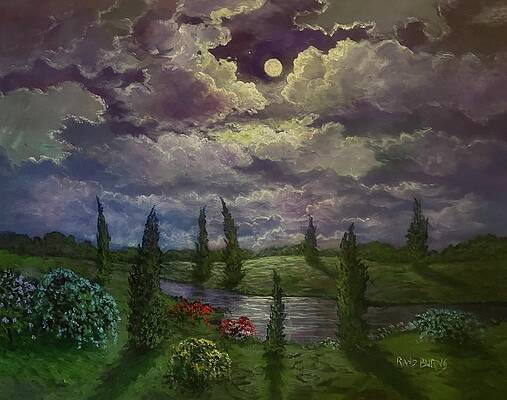This is a color painting executed with acrylics, depicting a serene nighttime outdoor scene. The sky, adorned with an array of fluffy, well-defined clouds, reveals only small patches of the dark bluish-purple night sky. A round full moon captures the viewer's eye, prominently centered in a gap among the clouds. Below, the landscape features a bright green field with Italian cypress trees lining a path, and an assortment of wispy and flowery bushes. The field is interspersed with red wildflowers adding vibrant splashes of color. Additionally, a river or small pond meanders through the terrain, flanked by grassy areas and a variety of flowering bushes. These bushes showcase a rainbow of blooms: white, pink, red, and yellow, further enriching the scene’s tranquil beauty.